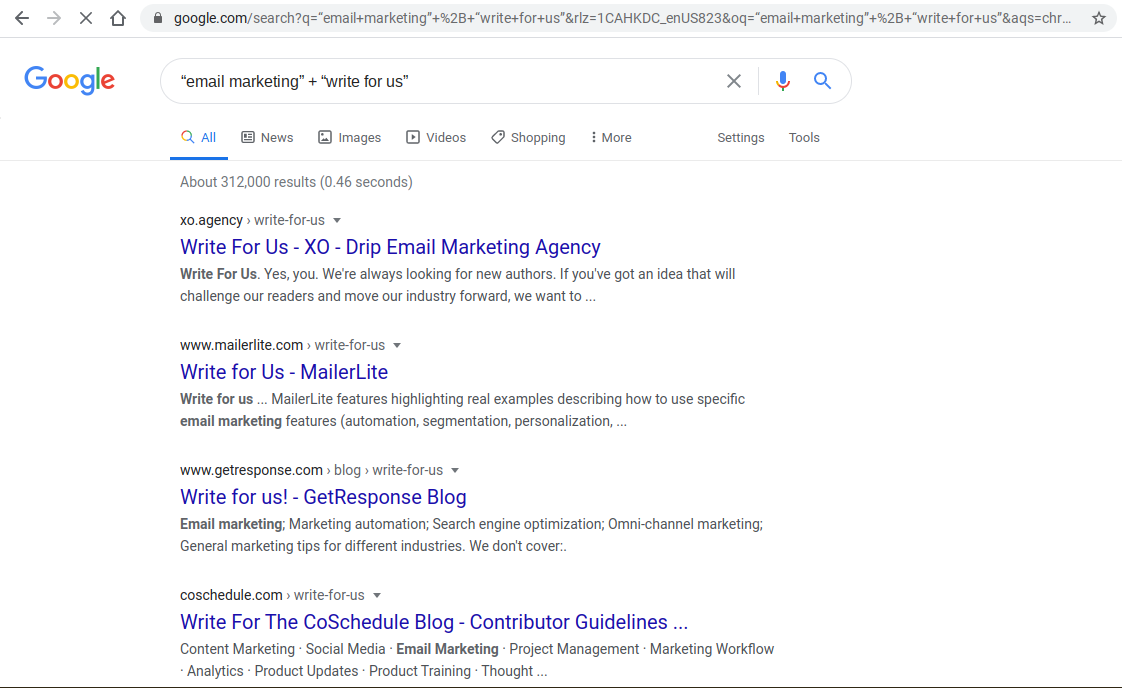The image captures a computer screen displaying a Google search results page. At the very top, a browser URL bar shows the address "google.com/search?" followed by the rest of the search term parameters. To the left of the URL bar are navigation icons including left and right arrows, a close (X) button, and a home symbol.

Below the URL bar, the familiar Google logo is prominently displayed. The search box contains the query "email marketing" + "write for us", and to its right are the icons for clearing the search (X), voice search (microphone), and initiating the search (magnifying glass). Beneath the search box, a menu bar features various search categories: All, News, Images, Videos, Shopping, More, Settings, and Tools. The "All" category is highlighted in blue.

Further down, the page indicates that there are approximately 312,000 results found in 0.46 seconds. The search results are listed below this notification. The first result includes the URL "XO.agency" with the title "Write for Us - XO - Drip Email Marketing Agency" in bold blue text. The description beneath reads: "Write for us. Yes, you. We’re always looking for new authors. If you’ve got an idea that will challenge our readers and move our industry forward, we want to..."

The second result follows a similar format, with the URL "www.mailerlite.com", the title "Write for Us - MailerLite" in blue, and a description mentioning how MailerLite features highlight real examples of using specific email marketing features such as automation, segmentation, and personalization.

There are two additional entries listed in the same structure. The bottom of the screen is marked by a dark black line. The background of the entire image is white, providing a clean and simple layout typical of Google's search results interface.